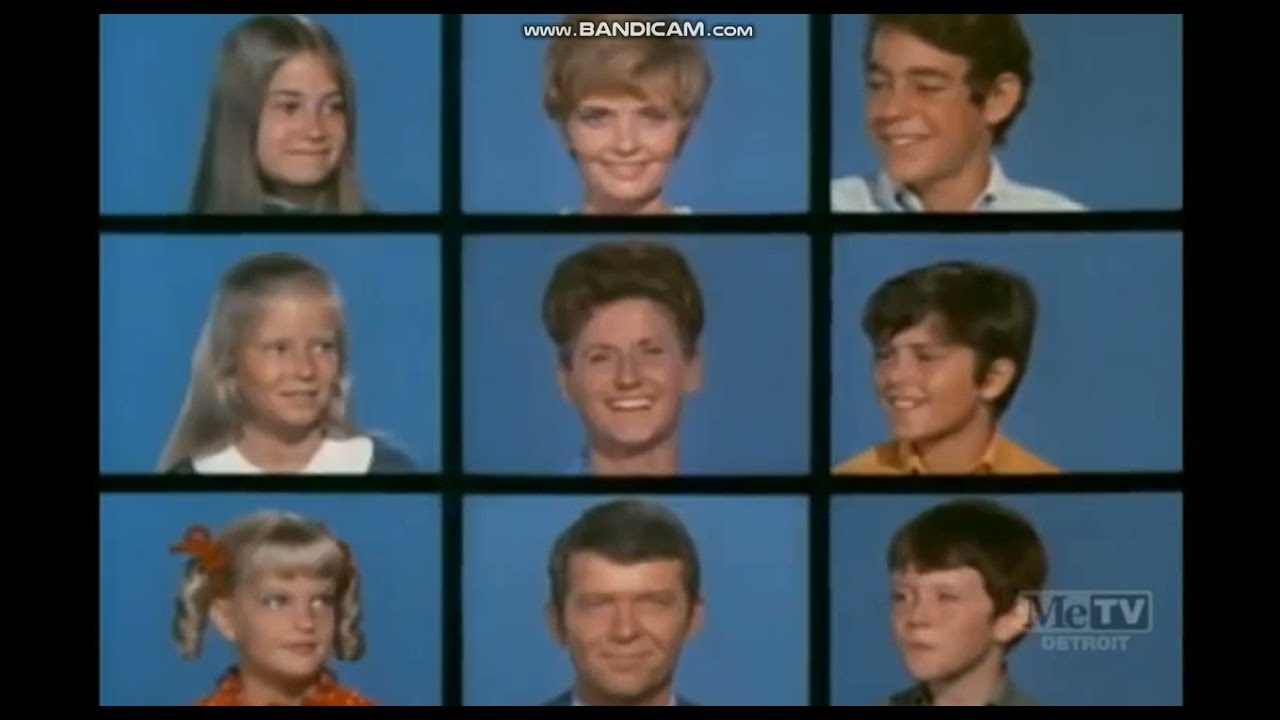This image is a classic still shot from the television show "The Brady Bunch." The entire image comprises nine blue squares arranged in a 3x3 grid, each containing a headshot of the main characters, set against a black background with black lines dividing the squares. Starting from the top row, from left to right: Marsha, the eldest blonde daughter; the mother, Carol; and Greg, the eldest son. In the middle row, from left to right: Jan, the middle daughter; Alice, the family housekeeper or nanny centrally positioned; and Peter, the middle son. The bottom row, from left to right: Cindy, the youngest daughter; Mike, the father; and Bobby, the youngest son. At the very top of the image, in the center, is the watermark "www.bandicam.com," while the lower right corner of Bobby's square has the text "Me TV Detroit."